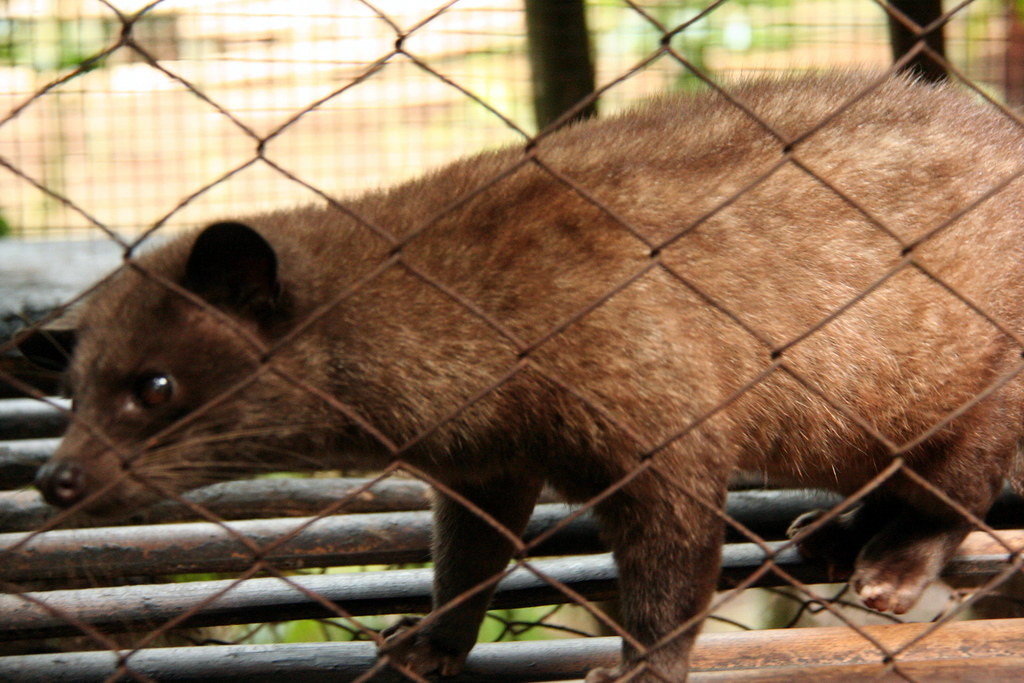This horizontally aligned rectangular photograph captures a small, fuzzy brown animal resembling a mongoose or wolverine inside an enclosure. The creature, with its short legs and long body, has a solid medium to dark brown fur coat, a face similar to that of a dog, and prominent pointed ears. It features large round brown eyes, a black nose, and noticeable whiskers protruding from its snout. The animal, standing on a wooden rod platform, is facing towards the left, appearing to gaze at something outside the frame. Its claws and toes are clearly visible. In the foreground, a rusted wire fence partially obstructs the view, while behind the animal, rusted black or dark gray bars add depth to the scene. The background is blurred, showing more wire fencing affixed to a couple of wooden posts at the top of the picture, hinting at daylight outside the enclosure.